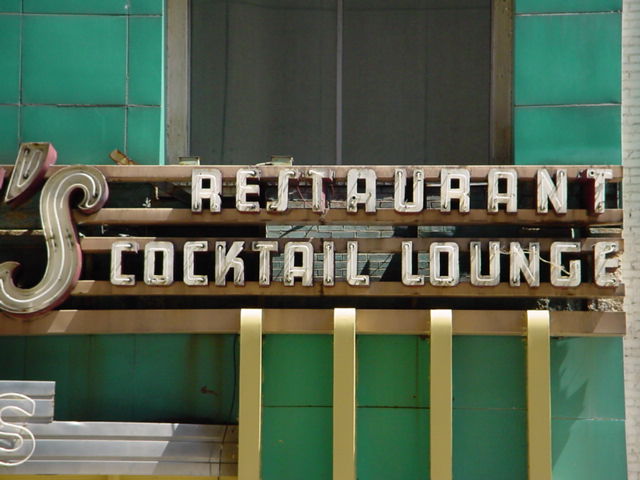This photograph captures a vintage sign for an old cocktail lounge, evoking a sense of bygone elegance. The sign, with a slightly tarnished gold and off-white color scheme, is affixed to a turquoise tile surface characterized by visible, dirty grout. Above the sign, there is a window, hinting at the building's interior. The sign itself is inscribed with the words “Restaurant Cocktail Lounge” in an off-white font. To the right side of this sign, a partially visible ‘S’ suggests another sign, though its full message remains obscured. Below the main sign, three vertical metal strips descend along the building’s facade, which includes a white adjacent surface. Another ‘S,’ likely part of a different sign, appears on this white surface, adding to the layered aesthetic of the scene.